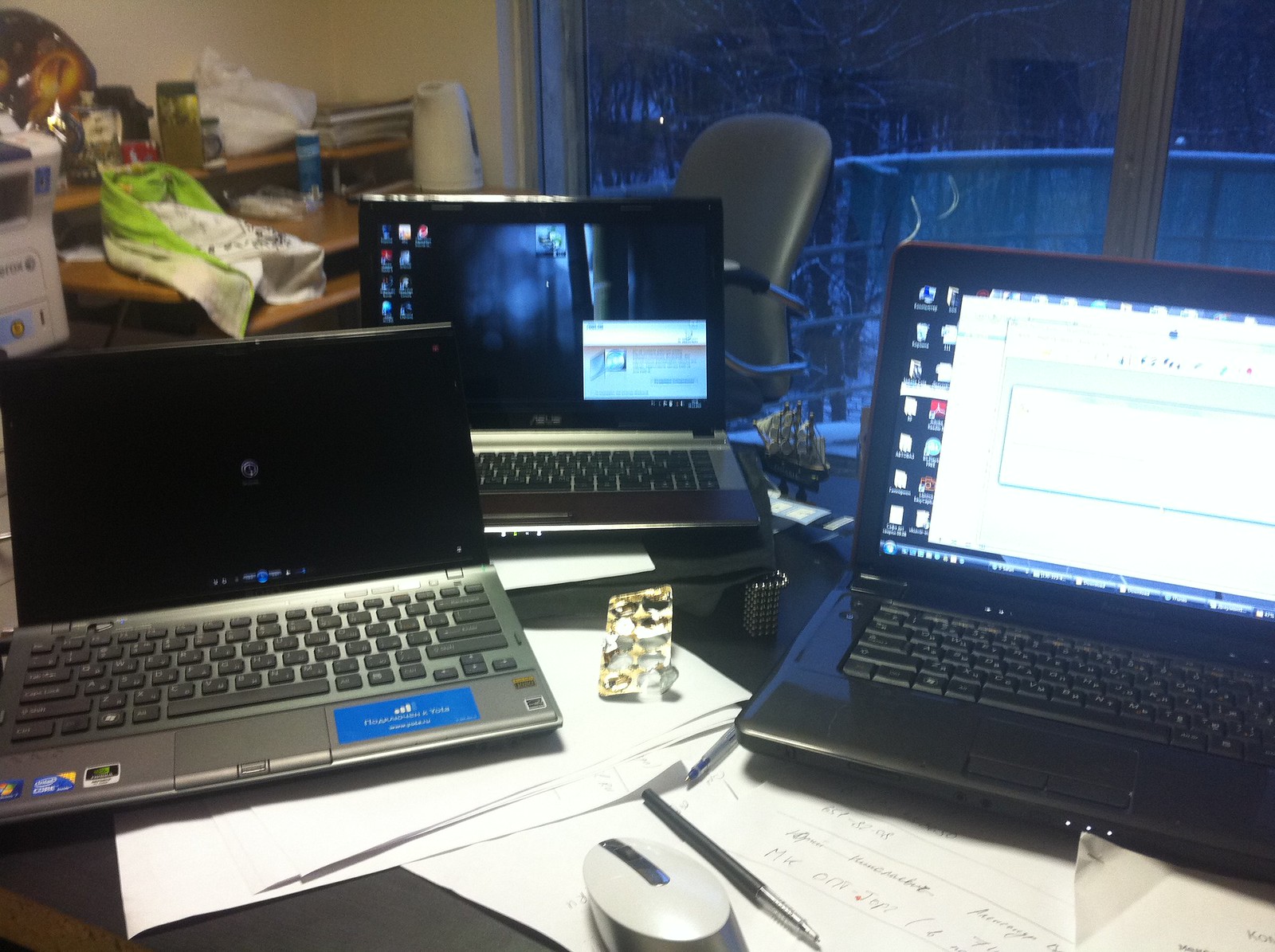In a cluttered office setting, three laptops are arranged in a wide triangle formation on a desk. The left laptop, which is off, has a black screen, silver base, and a dark gray keyboard, as well as various stickers. The middle laptop, which is turned on, displays a screensaver along with a Windows update box in the lower right corner. The right laptop, actively in use, shows multiple open windows and icons on its white screen, with a black keyboard and border. Sitting on the desk in the foreground, there's an assortment of papers, a black pen with a silver point, a silver mouse with a black clicker, and two pens. The background reveals further clutter, including a messy wooden desk to the left cluttered with a roll of paper towels and miscellaneous items, a printer, magazines, a green coffee cup, and a green and white scarf. An air purifier or humidifier with a white and blue design stands in the corner. To the right, a large window showcases a snowy exterior with trees and railings visible. An office chair is positioned nearby, and next to the mouse, there appears to be packaging from medication, now empty.